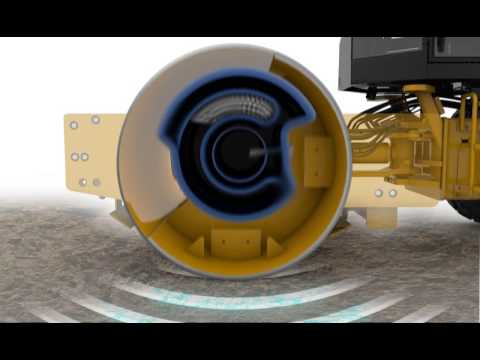The image is a horizontally oriented rectangle with black bars at the top and bottom. The background transitions from pure white at the top to a muddled gray at the bottom. Radiating from the lower portion are slightly translucent, white light arches. Centrally positioned is a circular piece of yellow machinery, possibly metal, encircled by a blue, C-shaped component that looks like plastic. This central structure somewhat resembles a brake drum but without the inner parts. Behind this assembly is a yellow structure that seems to resemble a train axle, contributing to the industrial feel of the scene. To the right of the machinery, there is a black box-like structure which might be part of the equipment or machinery, with a tire visible in the background. The overall composition has an almost unworldly appearance.